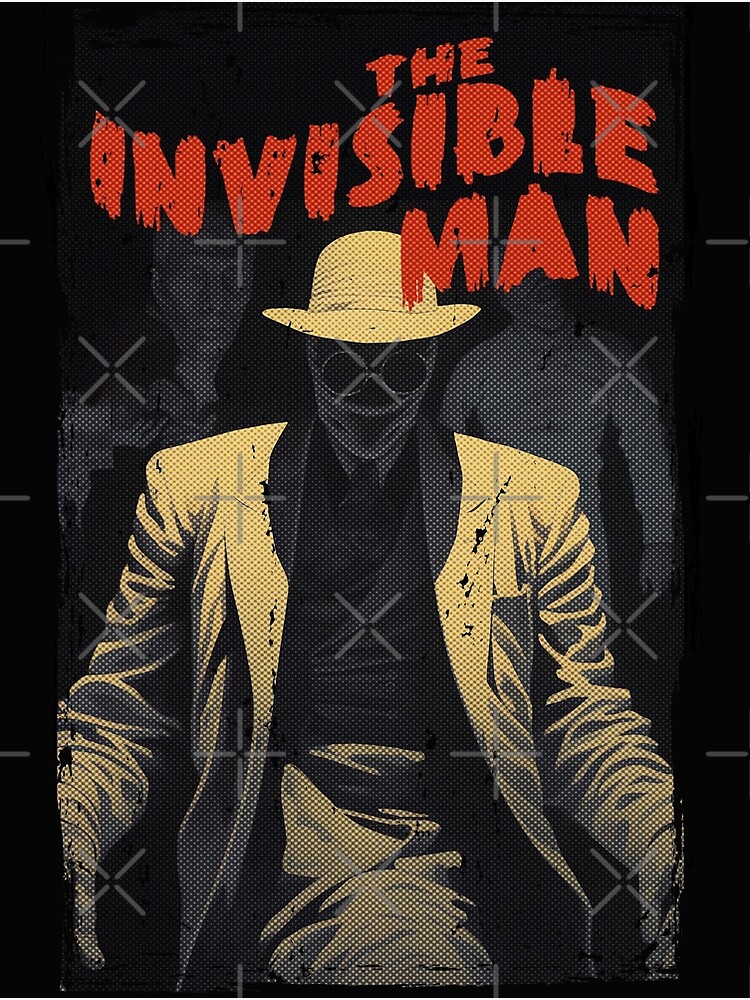This is a vintage movie poster for "The Invisible Man," intricately detailed and executed in a pixelated texture with a black background and bordered in black. At the top of the poster, the movie title "The Invisible Man" is written in eerie, blood-like red letters that look scribbled. Dominating the center of the image is the focal point: a man with a white hat featuring a wide brim, a mask with dark black eyes and a black triangle nose, dressed in an all-white suit with white pants and gloves. His hands rest on what appears to be armrests, and his figure is somewhat opaque, giving him an unsettling, almost ghostly presence. In the background, barely visible, are two silhouettes—a man on the left in a indistinct pose and another on the right wearing a long-sleeve white shirt with his head cocked to the side. The poster also features white X watermarks across its front, adding to the vintage and mysterious aesthetic.